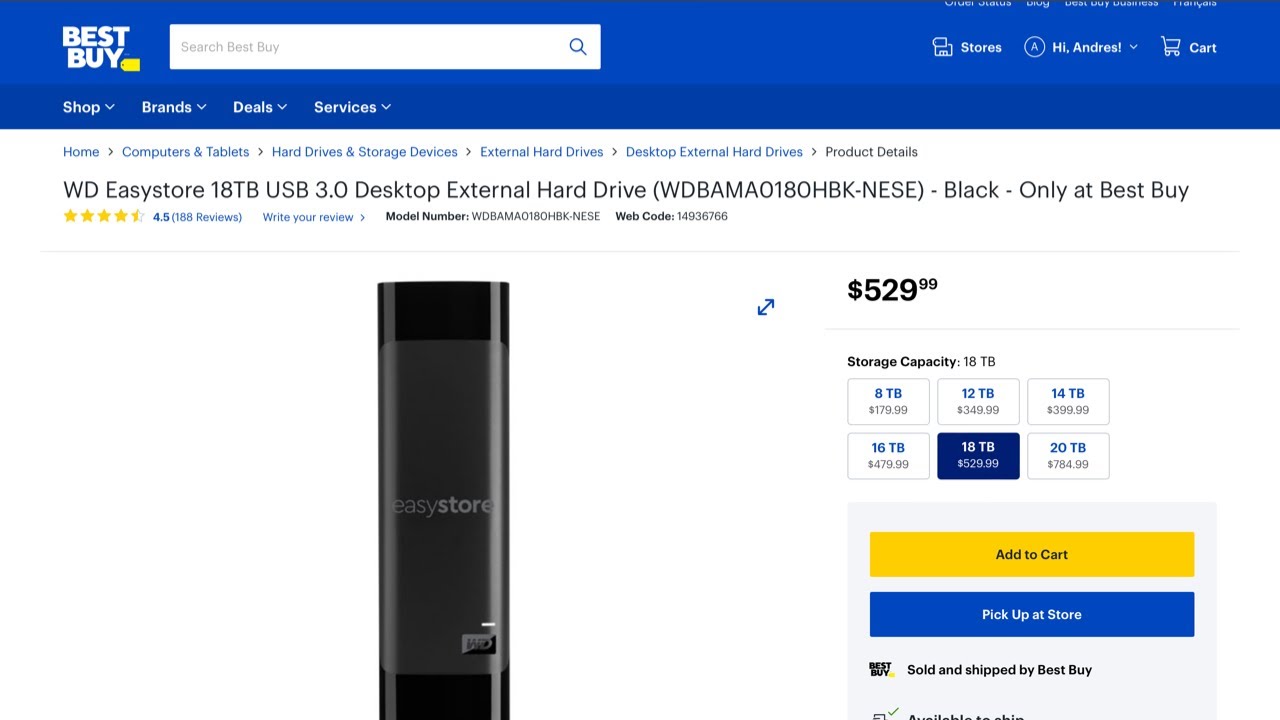This is a detailed descriptive caption for the image provided:

---

The image shows a product listing on the Best Buy website for the WD EasyStore 18TB USB 3.0 Desktop External Hard Drive. The product code displayed is WD BAM A0180HBK-NESE, and it is noted that the drive is available exclusively in black at Best Buy. The listing includes a model number, a web code, and a customer rating of 4.5 stars based on 188 reviews, with an option to write a review. The product is available in various storage capacities, ranging from 8TB to 20TB. Users can choose to add the item to their cart via a prominent yellow "Add to Cart" button or opt for store pickup using a blue "Pick Up at Store" button. The item description confirms that it is sold and shipped by Best Buy. Central to the webpage is the image of the sleek, black external hard drive with the "EasyStore" branding. The website's interface features a blue header with a white search bar, navigation sections for the store, a personalized greeting button labeled "Hi Andres" likely linking to the user's account, and a shopping cart icon.